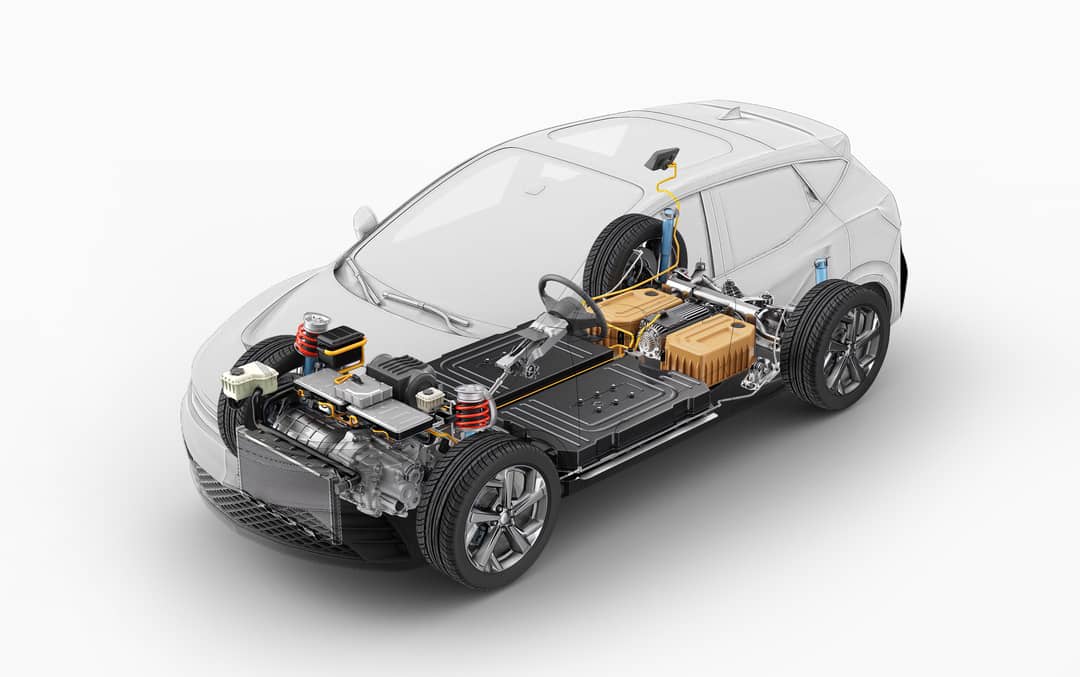This is a detailed, computerized cutaway diagram of a small SUV, potentially created by a car manufacturer to illustrate the advanced technology and infrastructure within the vehicle. The body of the car is rendered almost fully transparent, providing a clear view of its internal components. The SUV appears to be an electric vehicle, with prominent rectangular, light tan battery cells located behind the front seats. The image extensively highlights various mechanical elements such as the wheels, axles, and springs, as well as critical hardware including the engine block, radiator, gas tank, oil tank, brake fluid reservoir, and shocks. The car itself has no identifying brand, model, or year information, suggesting it is meant for demonstration or educational purposes, possibly part of a press release or a manufacturer’s promotional material.